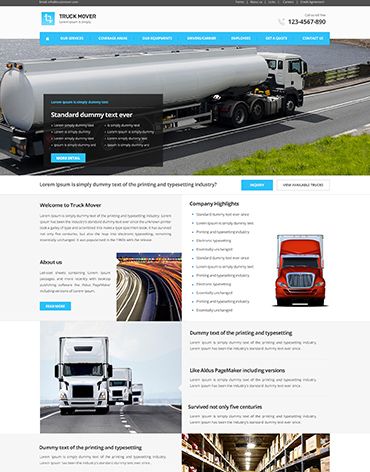This is a screenshot of a trucking website template. At the top left corner, the name of the website, "Truck Mover," is displayed in black font. Adjacent to the name is a blue square icon featuring a white circle. On the upper right corner, there's a placeholder phone number: 123-456-7890. Beneath the header, there's a blue navigation bar with clickable white text options.

The main section displays an image of a silver gas tank truck with a white cab. Overlaying this picture, there's a small black menu with white font that reads "Standard Dummy Text." The screenshot appears to be a demo of a website template being showcased, likely for promoting a web design subscription service aimed at helping users create similar trucking websites.